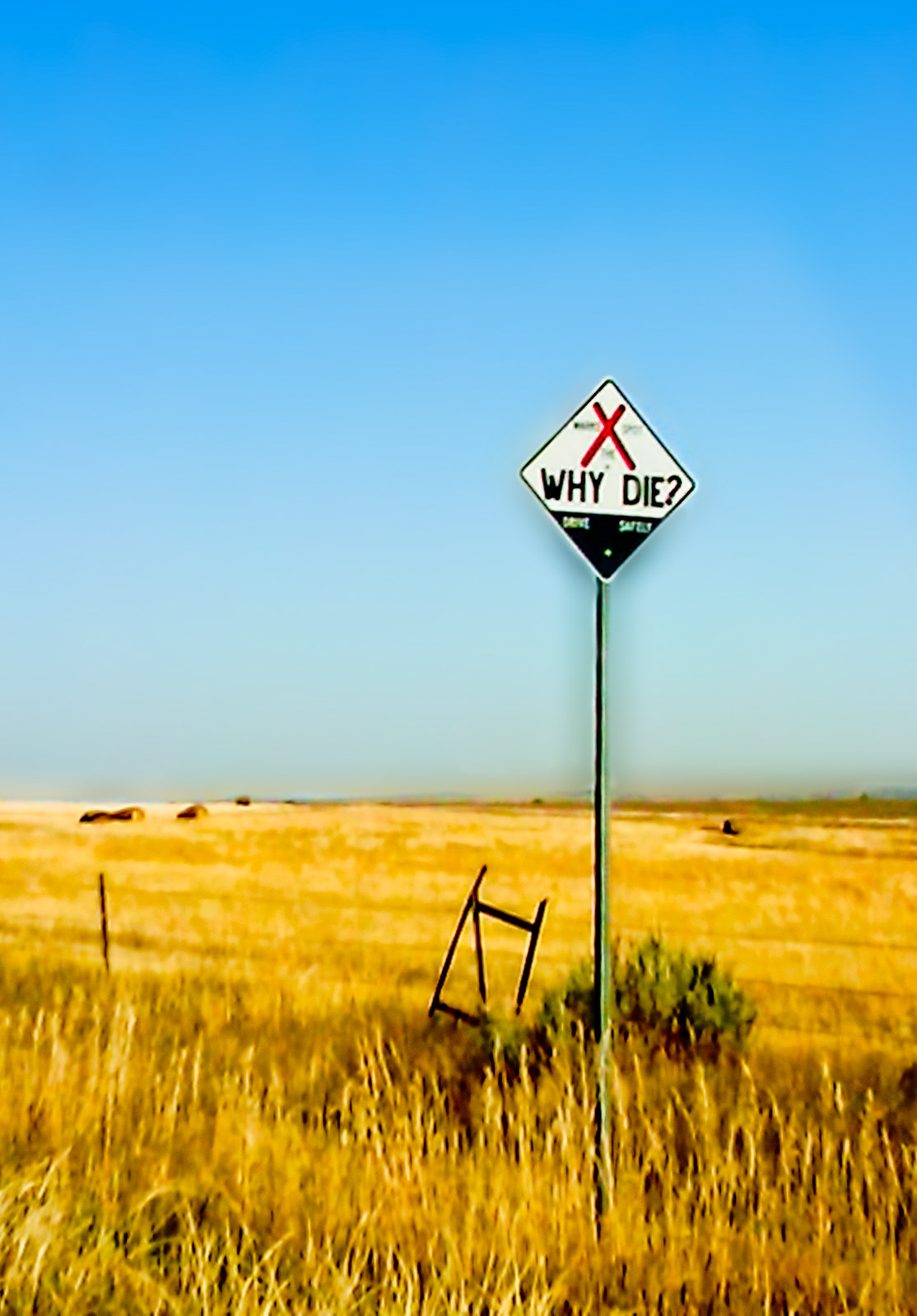This image features an unusual traffic sign placed on a long, thin pole that appears green. The sign itself is diamond-shaped and prominently displays a large black "X" at the top. Below the "X," in bold black font, the sign reads "Y-Die" against a white background. The bottom corner of the diamond is marked in black with additional white lettering. The photograph has a blurred quality, with fuzzy edges and an overall lack of detail, suggesting the possibility of a photographic filter or AI generation. In the backdrop, there is a serene field of golden wheat that stretches out under a sky, which transitions from a deep blue at the top to a lighter blue near the horizon.